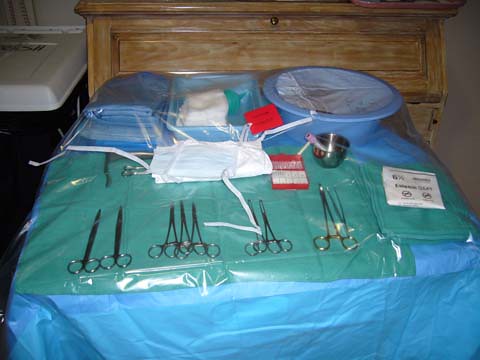This photograph, likely taken with a cell phone in poor indoor lighting, depicts a meticulously organized surgical prep setup on a light blue plastic-covered tabletop. The central focus is the array of surgical instruments, including eight pairs of scissors or hemostats, arranged on a green cloth. A single pair of tweezers is also present among the tools. In the middle of the table, a stack of white paper masks and another clear bag containing blue pads are visible. A small square tray, possibly holding gauze, and a blue bowl covered in plastic are located towards the upper right of the setup. There's also a shiny chrome cup filled with an unspecified content. Behind this array of tools and supplies stands a brown wooden surface, possibly the face of a chest of drawers or a headboard. To the left, a white cover, perhaps belonging to a black container, is partially visible. The well-ordered arrangement underscores the preparation for a surgical procedure.